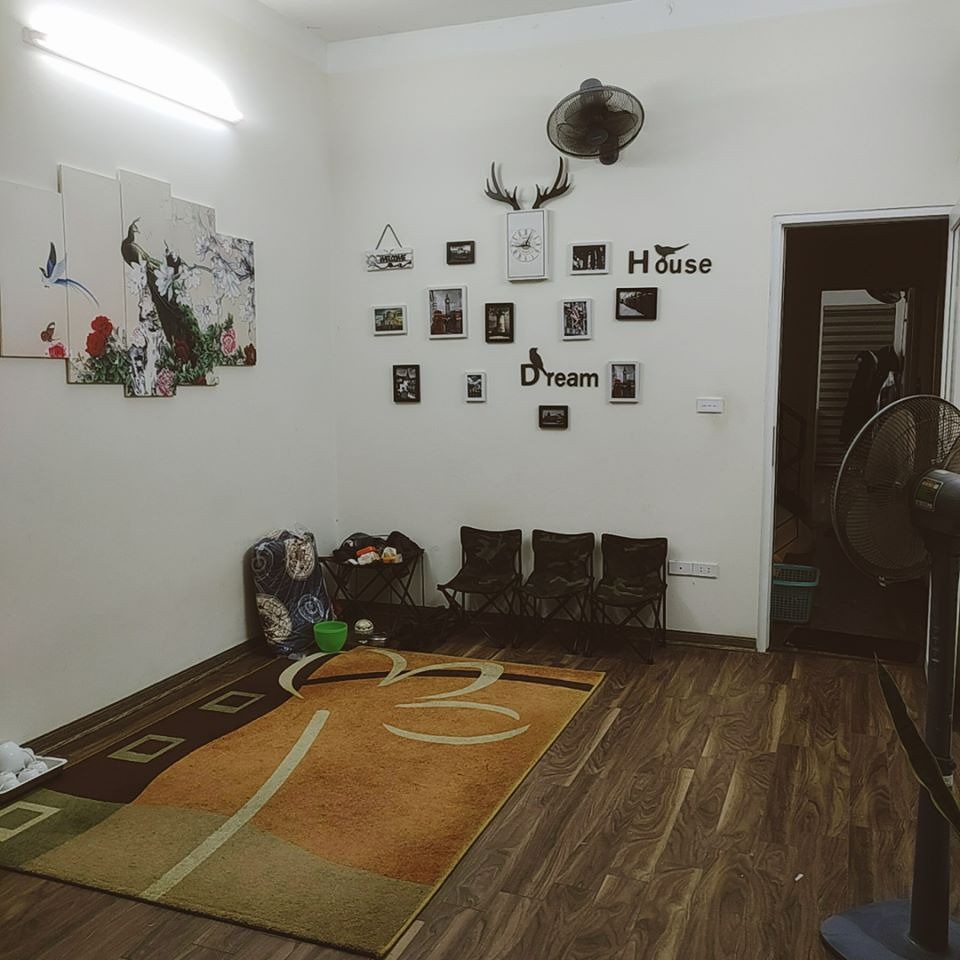The image showcases a stark white-walled room with very little furniture, likely a part of a house. A focal point on the left wall is a collage of five nature-themed pictures with a floral design, each framed in a white background. Further along the back wall, a collection of various framed black and white photos, a clock with antlers, and the words "DREAM" and "HOUSE" add to the eclectic décor, highlighted by small birds attached to the letters. A black oscillating fan is mounted high up on the back wall. The room features medium brown wooden plank flooring, partially covered by a tri-colored rug in browns and greens with an artsy pattern. There are three children's-sized folding chairs set up against the walls and a fourth camping chair in the corner. Additional elements in the room include a door with a mirror and a green basket leading into another space. A bright fluorescent light illuminates the scene from above.